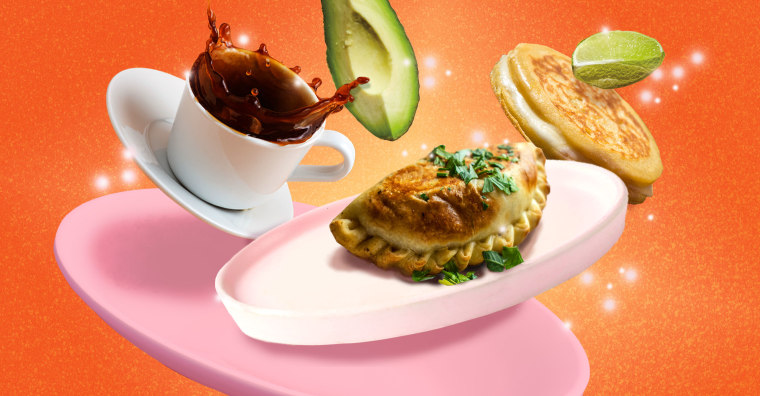This image captures a mesmerizing scene of food items suspended mid-air against a vivid orange background sprinkled with glowing white speckles. At the bottom left corner, a pink plate is diagonally positioned, contrasting with a lighter pink plate above it, angled in the opposite direction. Atop this lighter pink plate sits a perfectly crinkled, golden-brown calzone, garnished with fresh, bright green cilantro leaves. To the left of this plate, a white mug of black coffee splashes dramatically, spilling its contents sideways. Hovering to the right of the coffee is a cut avocado, with its exposed, creamy green flesh facing outward. Just to the right of the calzone is a thick pancake, and a wedge of lime sits enticingly above it. The interplay of these elements creates a dynamic and vibrant composition, as if the food is caught in an exhilarating moment of free fall.